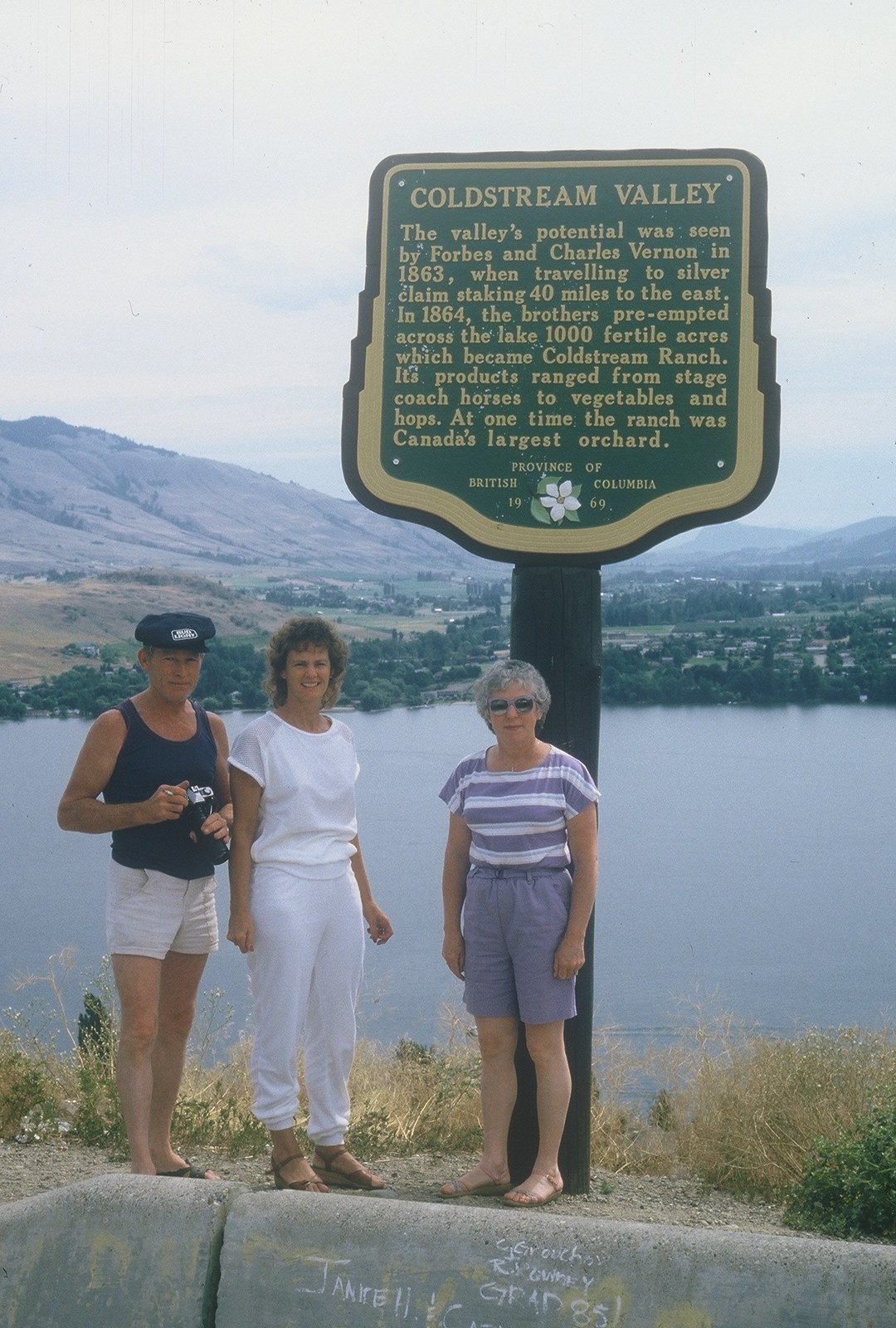In this detailed photograph, three older adults are standing on a grassy edge beside a river with a small cement area, adjacent to a tall, green signpost. The sign reads, "Gold Stream Valley. The greatest potential was seen by Forbes and Charles Berlin in 1863 when traveling to silver claims. By 1864, the brothers preempted 1,000 fertile acres across the lake, which became Cold Stream Ranch. Its products ranged from stagecoach horses to vegetables and hops, and at one time, the ranch was Canada's largest orchard. Province of British Columbia, 1969."

In the foreground, a man on the left wears a blue tank top, very short white shorts, and sandals, holding an old-school Nikon camera. He also dons a Bud Light hat. To his right, a woman dressed entirely in white—including her top and pants—wears brown wedge sandals and has long brown hair. Slightly to her right, an older woman stands, dressed in a purple and white striped t-shirt, gray high-waisted pants, and sunglasses.

In the background, there is a picturesque scene with a wide, open lake surrounded by a range of mountains, verdant green trees, and scattered houses at the mountain’s base, all under a broad sky. This appears to be a photo taken during a family trip or vacation, capturing a serene, natural landscape and the family's relaxed moment by the river.